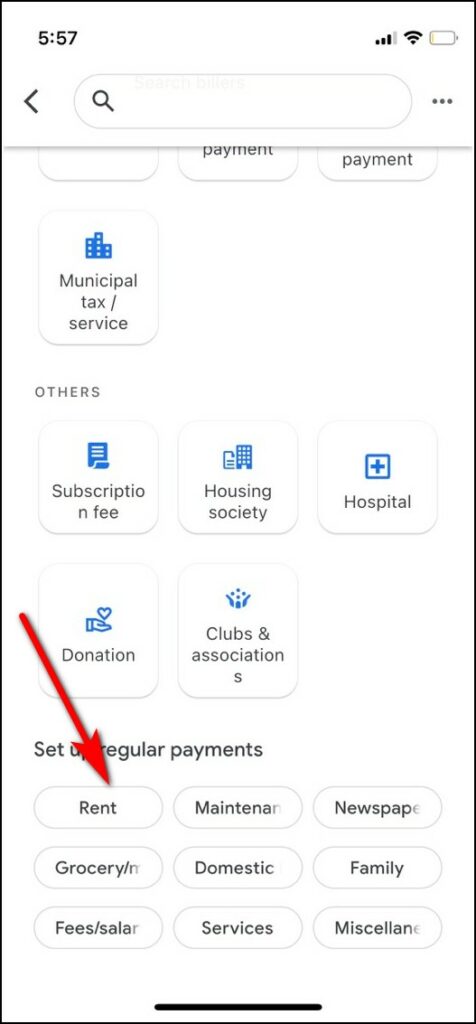This screenshot displays the interface of a payment organizer application. At the top, there is a white, pill-shaped search bar featuring a gray magnifying glass icon on the left side and a back arrow to its immediate left. Below the search bar, a series of white, square-shaped buttons are arranged, each adorned with blue icons representing different categories.

Directly under the search bar, there's a section labeled "Municipal Tax/Service" accompanied by a building icon. Following this is a section titled "Others" which includes:

- "Subscription Fee" with a document icon.
- "Housing Security" with a building icon.
- "Hospital" marked by a cross icon.
- "Donation" illustrated with a hand holding a heart icon.
- "Clubs and Associations" identified by a group icon.

Towards the bottom of the screen, the phrase "Set up regular payments" is prominently displayed. A red arrow points downward to highlight the first button labeled "Rent." Below this instruction, there are nine pill-shaped buttons arranged in rows of three. These buttons likely facilitate various regular payment setups within the app.